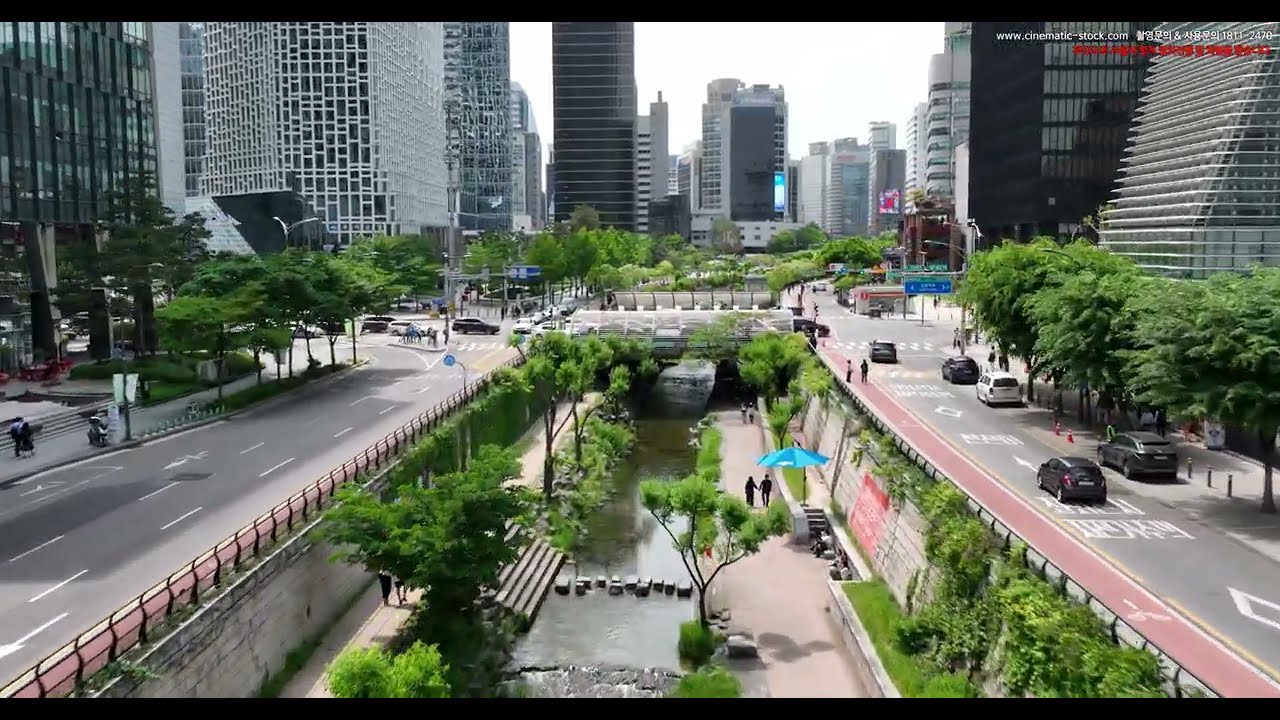This detailed landscape image depicts a bustling city during the middle of the day, featuring a striking juxtaposition of natural and urban elements. Dominating the center of the image is a body of water, likely a river, flanked by sidewalks and populated by small trees approximately 20 feet tall. The river is traversed by a bridge and lined with handrails, providing a safety barrier.

On either side of the waterway, multi-lane highways carry a steady stream of cars toward and away from the dense cityscape, which is adorned with numerous skyscrapers and large buildings. Sidewalks on both sides of these roads are dotted with some vegetation and occupied by people walking along the paths. 

In the foreground, near the river, a few individuals can be seen strolling, while a tent is pitched closer to the water. The vibrant color palette includes shades of gray, white, tan, green, brown, black, red, blue, and silver, enhancing the urban scenery. The composition is captured within a letterbox frame, with visible bars at the top and bottom, and includes some text in the upper right corner: "www.cinematicstock.com" along with Chinese characters and some red writing underneath. This image beautifully showcases the dynamic interplay between the city's infrastructure and the natural landscape.